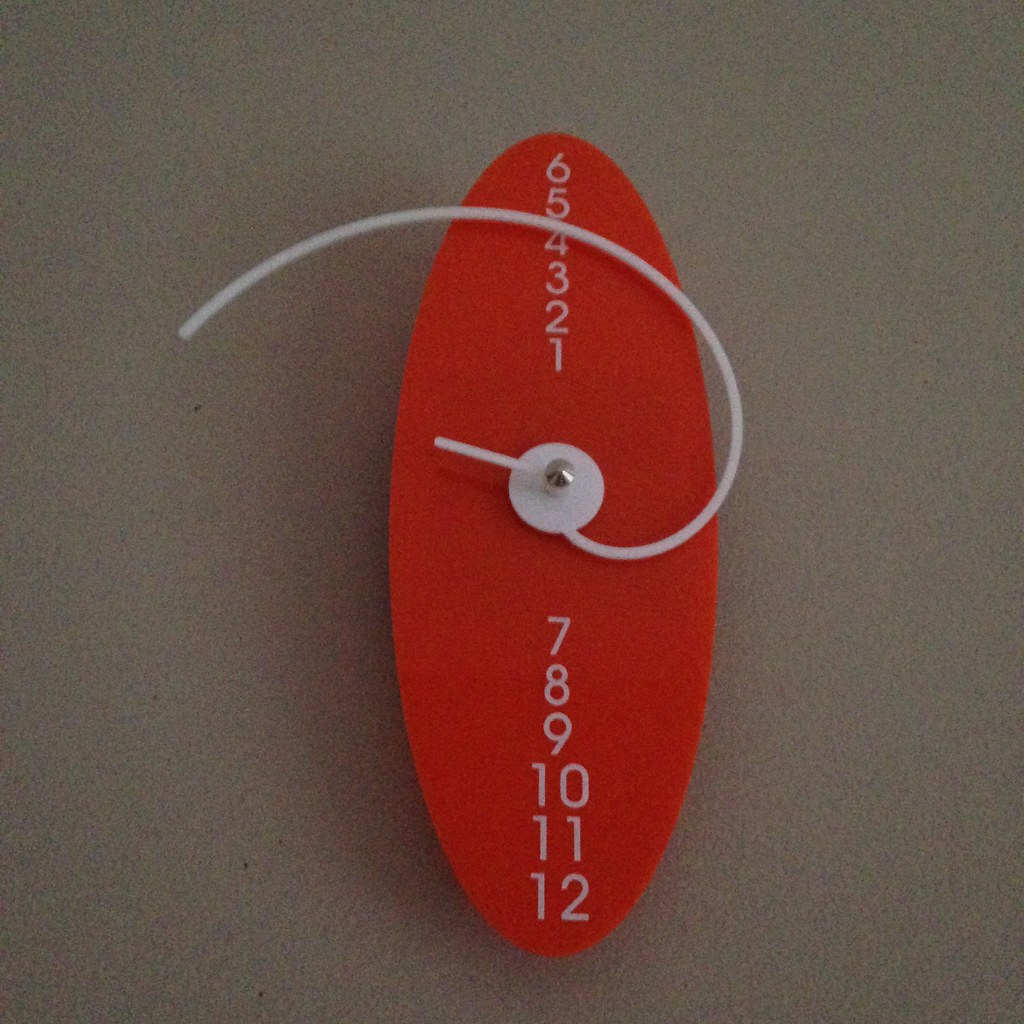The image features a gray background with a prominent red, elongated oval in the center. The oval stretches horizontally and isn't perfectly symmetrical, giving it a somewhat straightened appearance. Central to the oval is a curvy, white clock hand that appears to draw inspiration from an artistic clock design. Surrounding this clock hand are numbers, also in white, arranged sequentially in a circular manner, starting with '1' at the top middle and proceeding clockwise to '12' at the bottom middle. The arrangement of the numbers and the curvature of the clock hand give the image a modern, abstract feel, making it resemble an avant-garde timepiece.